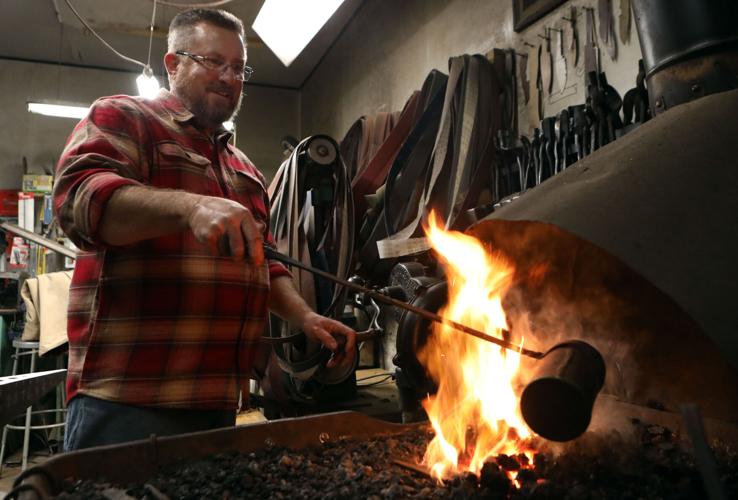In this photograph, a middle-aged white man with glasses and a light beard, dressed in a red, black, and white plaid button-down shirt and jeans, stands on the left side of an apparent workshop or garage, surrounded by cluttered tools and equipment, including knives on a rack and shelf, various hoses, and belts. He has dark hair and light skin and is smiling as he engages in some form of barbecuing or hot work. The main focus of the image is the large charcoal grill in front of him, where he is using a long-handled tool with a small cylindrical cup at the end to pour something—possibly sauce or another liquid—onto the coals, which causes a dramatic burst of flames. The prominent flames capture the viewer's attention, highlighting the intensity of the heat and the activity.